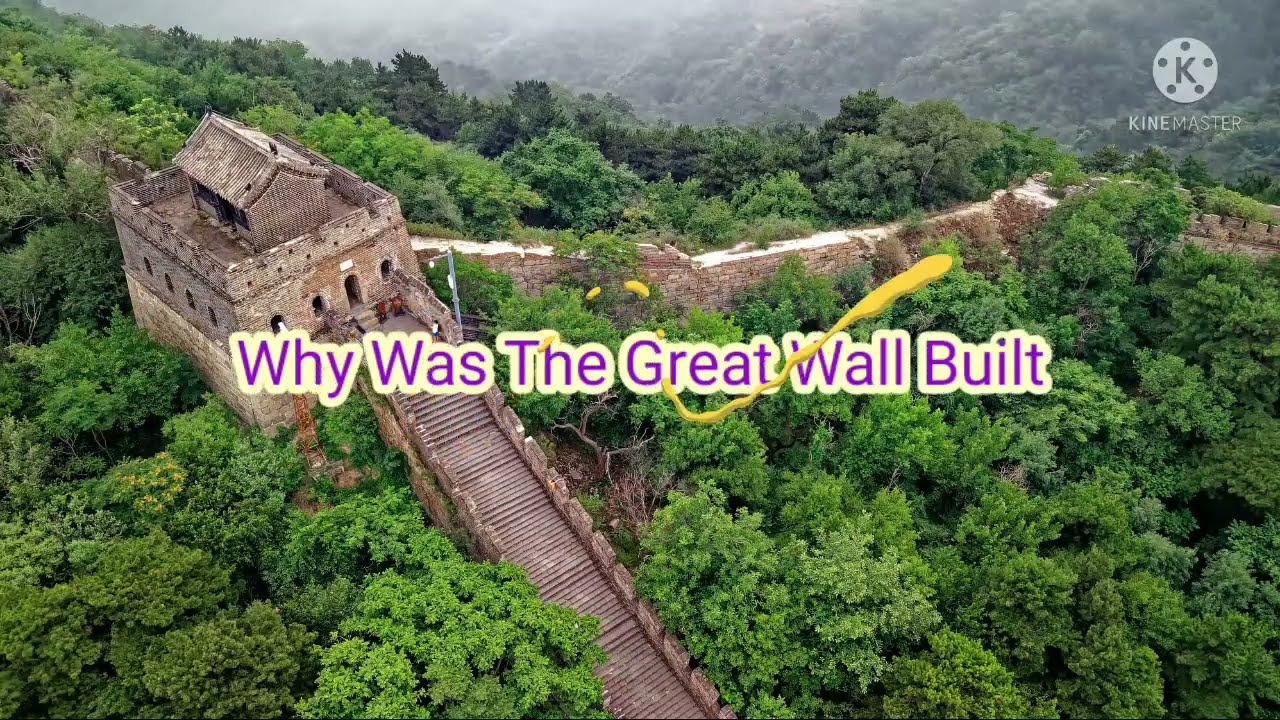The image depicts an outdoor view of the Great Wall of China, centered prominently. A text with a yellow glow and purple letters is overlaid, reading "Why Was the Great Wall Built?" with each word capitalized. A distinctive yellow loop decorates the text, starting behind it, swooping below the letters "GR" in "Great," and then arching up and across the "W" in "Wall."

At the forefront of the scene, a stone staircase extends upward, leading to a smaller structure that resembles a tower with four arches and a roof. This tower is connected to the main section of the wall, which continues to the right as a relatively smooth stretch of the fortification. The surrounding area is lush with vibrant green trees, which fill both the foreground and background. 

The distance is shrouded in a light fog, partially obscuring more trees and adding a misty, ethereal quality to the landscape. In the upper left corner of the image, a circle with five dots and a "K" in the center is visible, and below, the text "Klein Master" can be seen. On the upper right, there is another caption that reads "Keen Master."